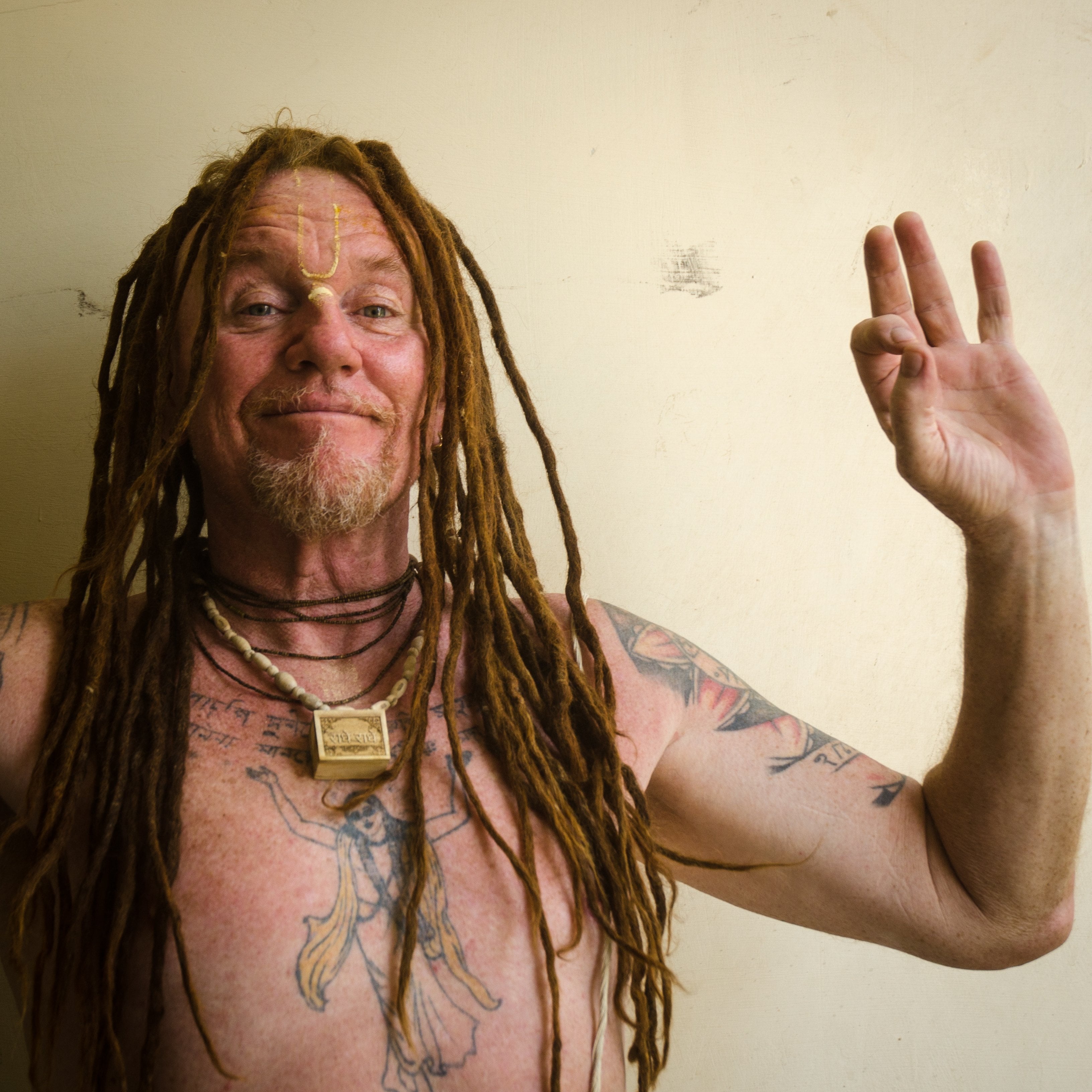In this image, we see a shirtless Caucasian man with a distinctive appearance. His face features bluish eyes and reddish brownish dreadlocks that hang down to his stomach. He has a small mustache and a white-and-yellow beard, both worn lightly, and blondish colored eyebrows. His skin has a somewhat reddish hue, and his forehead is notably wrinkled with a marking resembling a 'U.'

The man's body is adorned with various tattoos, including a prominent one on his chest of an Egyptian-looking woman with her arms raised, appearing to dance, and a large colorful tattoo on his left bicep. Around his neck, he wears multiple necklaces: dark brown, string-like chokers and a seashell necklace featuring a square box at its center.

He's smiling directly at the viewer and holding his left hand up in an "OK" gesture, with his thumb and index finger forming a circle and the other fingers fanned out. The background of the image is a light shaded yellow wall.